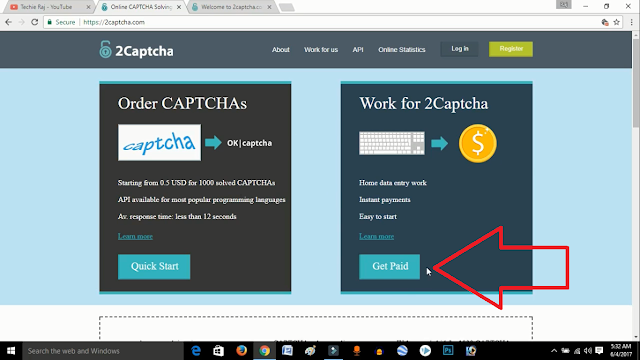The image is a screenshot of an open computer screen displaying several browser tabs. The focused tab is from the 2CAPTCHA website. The website's interface includes a blue navigation bar at the top with the 2CAPTCHA logo, which features an open lock icon. The navigation bar contains the following options: About, Work for Us, API, Online Statistics, and a Login button that is a slightly darker shade of blue. There is also a green button, though the text on it is partially obscured but likely reads "Register."

Below this navigation bar, the main section of the website is a large light blue area. Within this area are two prominently placed blue squares. The first square offers a service to "Order CAPTCHAs," providing examples and a "Quick Start" button for users who want to purchase CAPTCHA solutions. The second square, highlighted by a red arrow pointing towards a "Get Paid" button, is labeled "Work for 2CAPTCHA." This section appears to showcase how users can earn money by solving CAPTCHAs, indicated by an illustration of a computer and keyboard pointing towards cash. 

Additionally, there are two other browser tabs partially visible in the screenshot: one showing a YouTube page and another tab that is unreadable except for the partial title "Welcome to." However, the primary focus remains on the 2CAPTCHA tab.